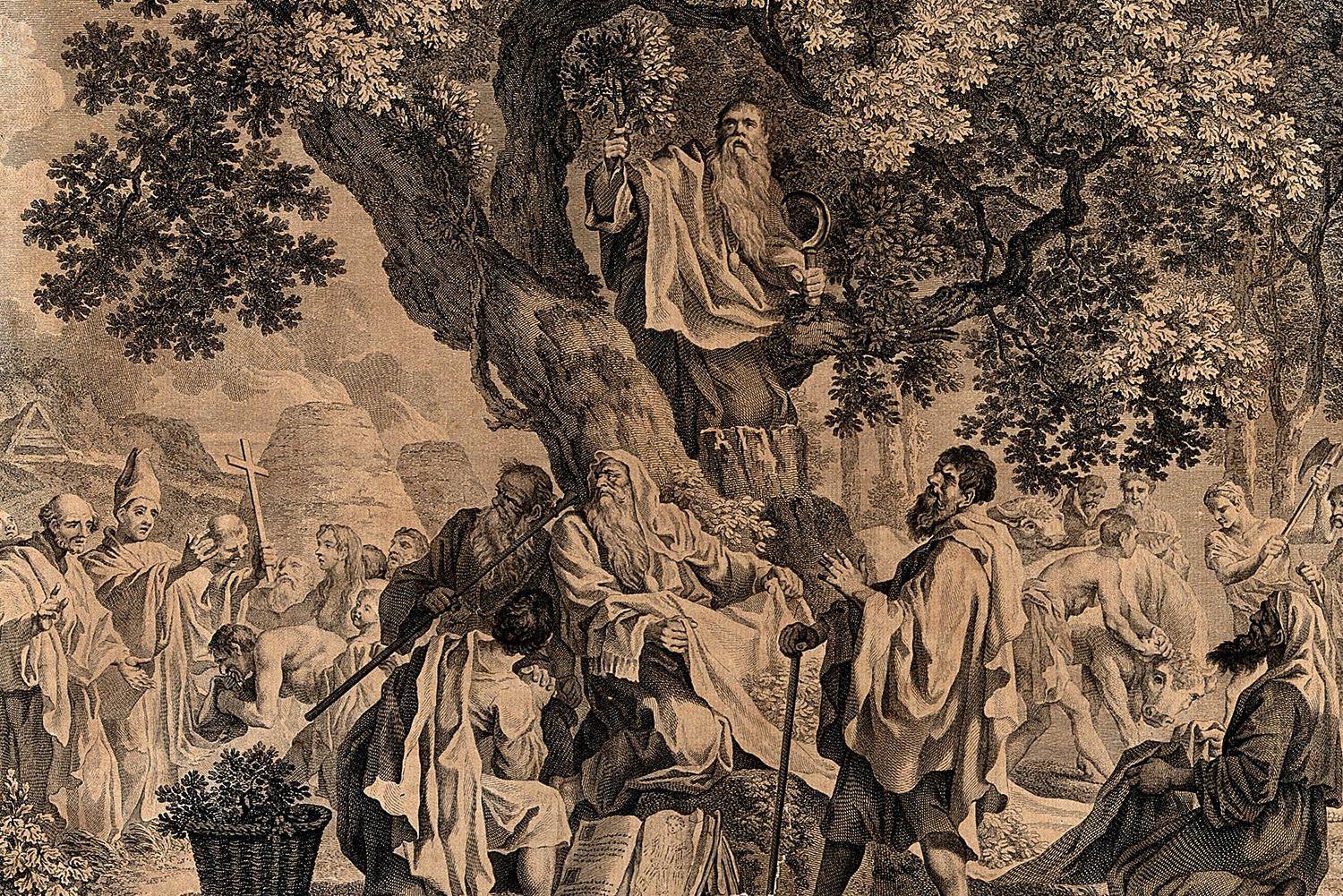This sepia-toned image, reminiscent of an old-time engraving, depicts a historical scene that appears to have religious and ceremonial undertones. At the center, a man with a long beard, clad in robes, is perched in a tree, holding a sickle and a branch from a small bush or tree. Surrounding him are various figures in ancient robes, suggesting a group from a past era, potentially the Crusades.

On the left, a priest is prominently featured, holding up a cross as a man kneels before him, seemingly kissing the hem of his robe. The scene is bustling with activity as numerous robed individuals gather around the tree, some directing their attention toward the priest.

A key detail to the right reveals a man gripping the horns of a bull or ox, poised to be slaughtered with an axe raised in the air. A basket containing green leaves is also visible, adding to the image's complexity. Various books and scrolls are scattered in the bottom foreground, hinting at the significance of knowledge or scripture in this assembly.

Overall, the painting gives an impression of a ritualistic or religious gathering with elements of sacrifice, devotion, and historical significance.